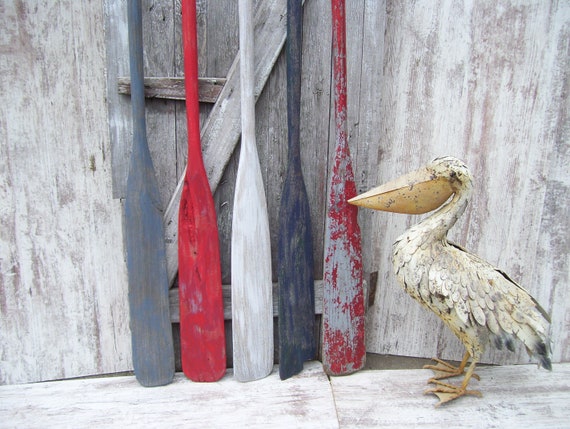The image showcases a rustic, aged wooden wall with faded white paint as its backdrop, against which five weathered rowing oars are displayed. From left to right, the oars are painted dark grey, red, white, and black with thin grey stripes, and another red oar with its paint worn off revealing a light grey base. The weathered oars are mounted on a white surface, supported by horizontal wooden bars at the bottom and near the handles. In front of these oars stands a large, statue-like pelican with a prominent closed beak, white feathers marred by black spots, particularly on the tail tips. The pelican's antiquated, slightly grimy appearance suggests it is an ornamental piece rather than a live bird, fitting into the decor that suggests an outdoor theme, potentially reminiscent of a quaint seaside restaurant or a rustic maritime setting.